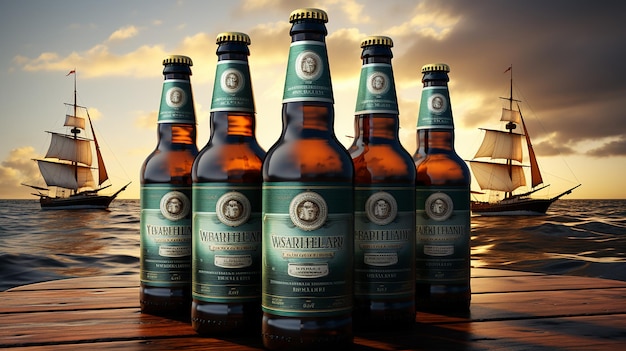This image is a wide artwork or advertisement showcasing a rustic scene with a nautical backdrop. In the foreground, there is a round, wooden table made of slats, stained a dark amber color. On the table, five amber-colored beer bottles, each adorned with green and black labels and bronze bottle caps, are arranged in a triangular formation. The text on the labels is illegible, suggesting that this might be AI-generated artwork. Behind the table stretches a dark, ominous ocean under a partially cloudy sky. On both the left and right, the horizon features majestic sailboats reminiscent of old pirate ships, adding a sense of adventure and historical charm to the scene. The lighting in the sky transitions from a foreboding gray on the right to a lighter blue with sunlight filtering through the clouds on the left, creating a dramatic and captivating atmosphere.